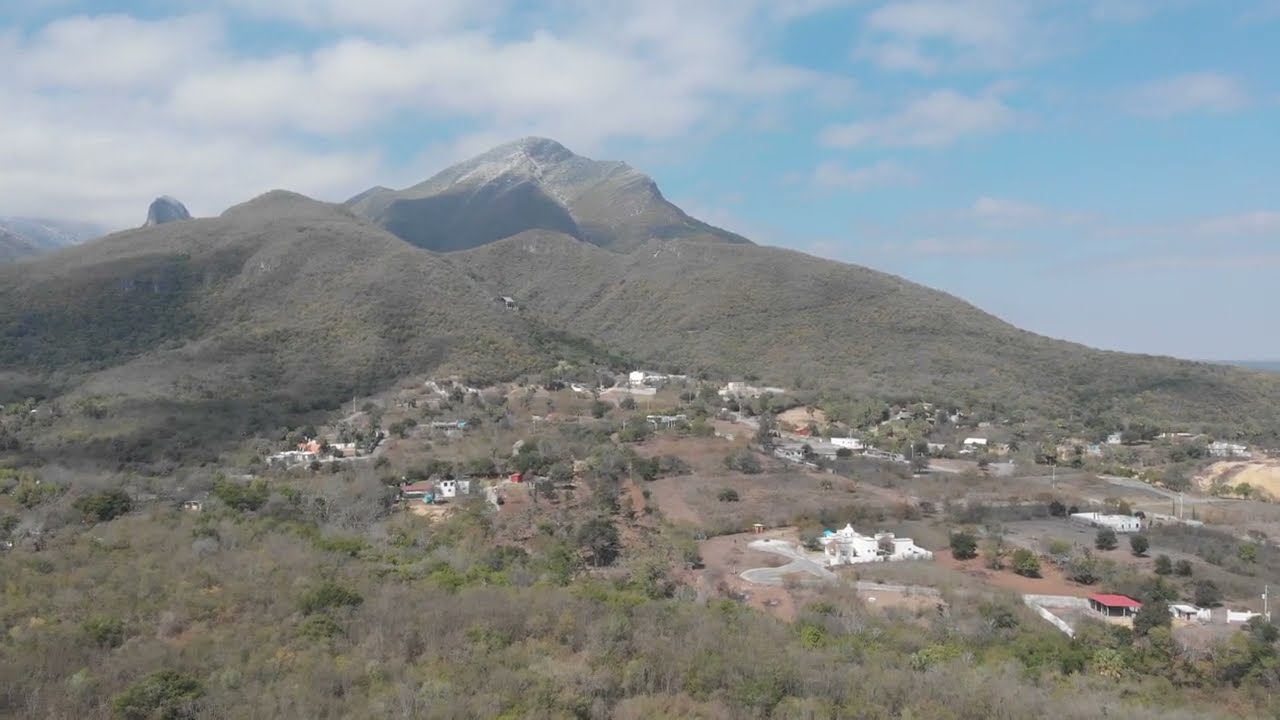The image shows a large hill with a small, scattered town nestled at its base. The sky is a light blue with sporadic white clouds, primarily concentrated on the left side. The hill itself is covered in a mix of brown and gray vegetation, with its tip a dark gray, suggesting a rough or rocky surface. In the distance, additional hills with varying vegetation can be seen. The town is composed of mostly white buildings, some topped with red roofs, creating a quaint and somewhat disorganized layout. There are a few paved roads winding through the town, many ending in round cul-de-sacs. In the foreground, treetops are visible, some appearing leafless, hinting at a late fall or early spring season. The area appears to include a park with walking paths and a few dilapidated buildings. The overall scene portrays a calm, semi-rural environment under a tranquil sky.